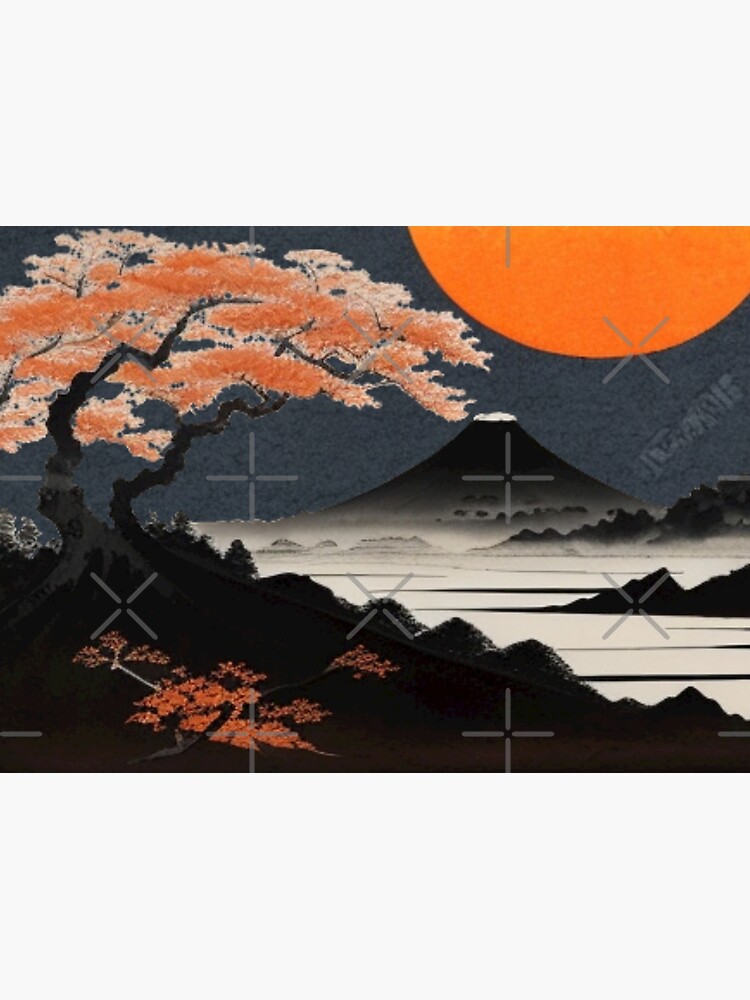This stylized, Japanese-inspired image features a captivating composition of elements. Dominating the foreground is a tree with a distinct, crooked trunk and limbs reminiscent of a bonsai, adorned with vibrant orange blossoms and foliage, which are scattered across the dark hillside. Surrounding this tree are lower vegetation with the same orange hues. From the bottom right, a series of mountains or hills ascend diagonally, veiled in a misty fog. In the backdrop, a prominent, smoothly curved volcano with a white cap rises elegantly, highlighted against a monochrome palette. A large, round orange orb—either the sun or moon—sits in the upper right corner, casting a warm glow over the scene. Throughout the image, there are intermittent pluses and X-like marks, adding an abstract touch, with what appears to be a signature on the left side. The blend of natural elements and abstract details creates a serene, yet dynamic visual experience.